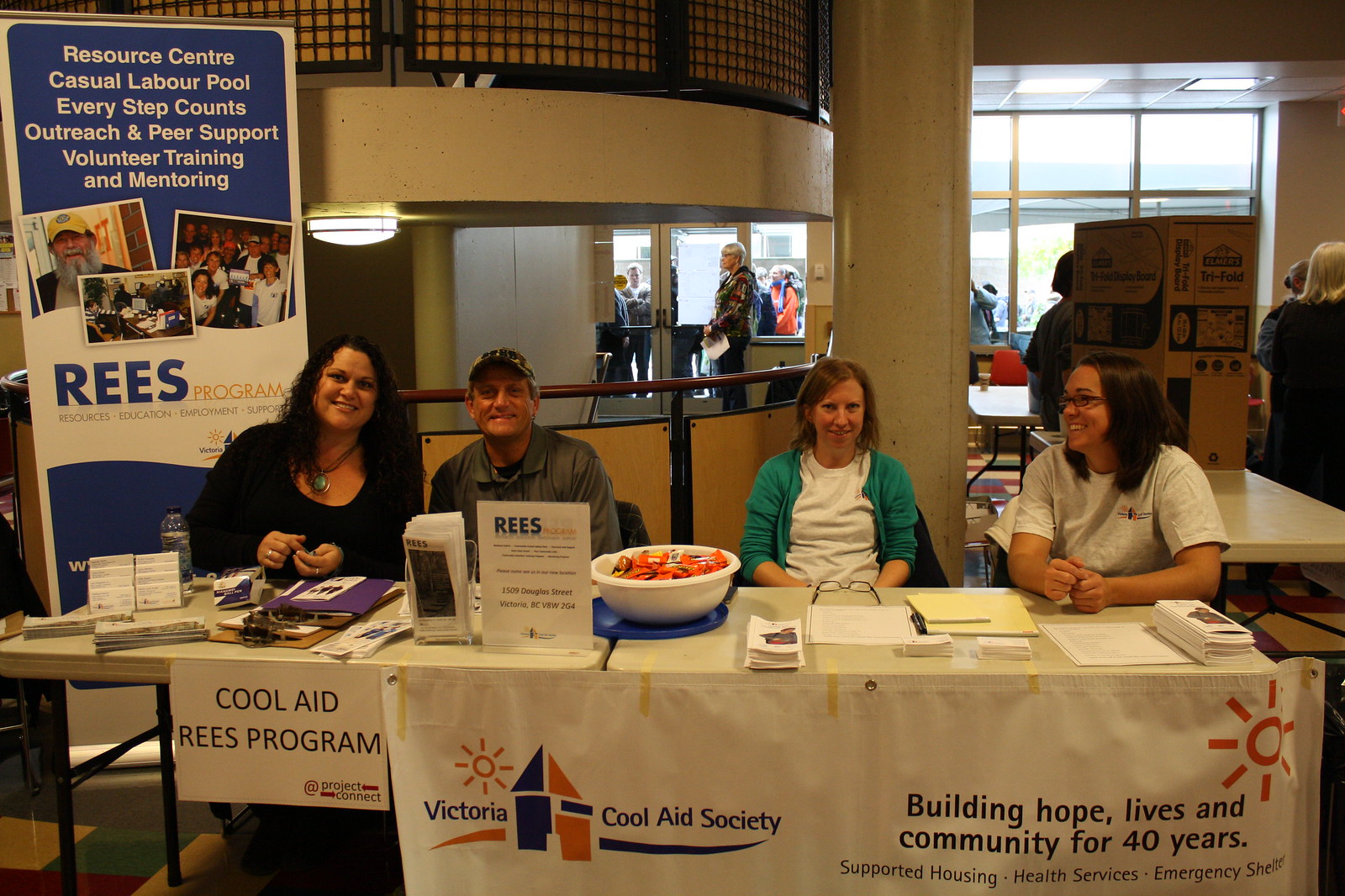This photo depicts an indoor setting, likely a resource center, captured in the middle of the day. At the forefront of the image is a long table, taped with a tarpaulin poster that reads "Victoria Cool Aid Society, Building Hope Lives and Community for 40 Years." The poster also features the REES Program, which stands for Resources, Education, Employment, Support.

The flooring is carpeted, adding to the venue's inviting atmosphere. At the table, situated centrally in the image, four people are seated, likely volunteers engaged in program activities. They are surrounded by various materials, including brochures, pamphlets, business cards, clipboards, and a bowl of candy, indicating a well-organized display aimed at informing and assisting visitors.

To the left of these volunteers, there is a sign reading "Resource Center Casual Labor Pool, Every Step Counts, Outreach and Peer Support, Volunteer Training and Mentoring," providing insights into the extensive services offered. Behind the table, an entryway with a glass door shows a woman standing at the entrance, with a crowd visible outside, suggesting a bustling environment and significant interest in the program.

The color palette of the scene includes shades of white, purple, orange, black, yellow, tan, brown, and blue, adding vibrancy to the detailed and informative setup.